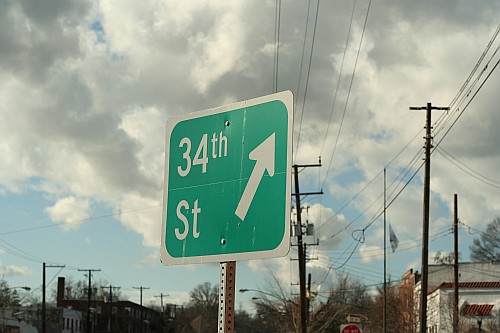In the center of the photograph, a rectangular green street sign with a white reflective border prominently displays "34th Street," with "34th" situated above "Street." To the right of the text, a large white arrow points upwards and to the right, suggesting a directional cue. The sign is affixed to a metal post. The background of the image is characterized by a partly cloudy sky, featuring both white and gray clouds with patches of blue visible. Numerous telephone poles and electric wires crisscross the sky, contributing to a busy, urban atmosphere.

In the lower right corner, a white two-level building is visible. Additional buildings can be seen on the left and right sides of the image. The scene is lightly dotted with trees, and various other signs and lampposts are scattered throughout, including a stop sign and a one-way sign. A flagpole bearing a mostly white flag at half mast is also visible, further adding to the detail in the background.